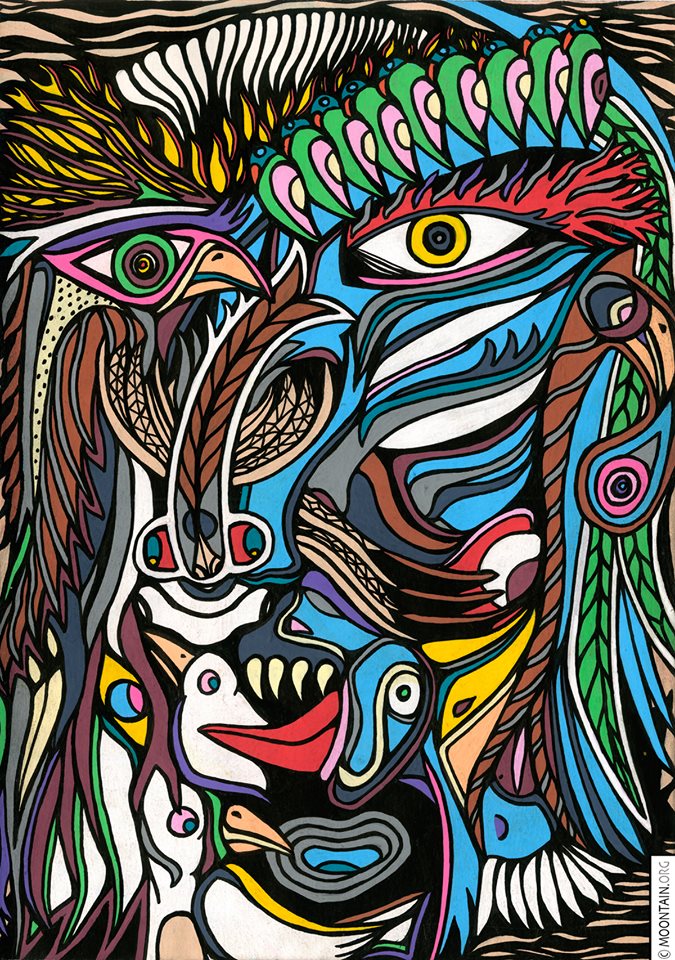The image presents a vivid, layered montage of animals and colors, evoking a sense of chaos and wonder. Dominated by avian forms and eyes outlined in vibrant colors, the scene transitions from feather-like patterns at the top, where birds and yellow flame-like shapes stand out. Central to the composition is a striking depiction of an eagle's yellow eye. Interwoven with red, blue, green, white, and yellow hues, the artwork features various creatures, including a blue snake with red and green accents and a bizarre blue creature with sharp teeth seemingly attacking a white bird at the bottom. This intricate tableau, reminiscent of Pacific Northwest totem designs, merges into a kaleidoscope of browns, blues, and greens, culminating in a mysterious signature at the bottom right: "Cappy Mountain dot O R I G." The artwork, a far-out yet groovy depiction of birds and animals, blurs the boundary between reality and abstract, offering an endlessly fascinating visual experience.